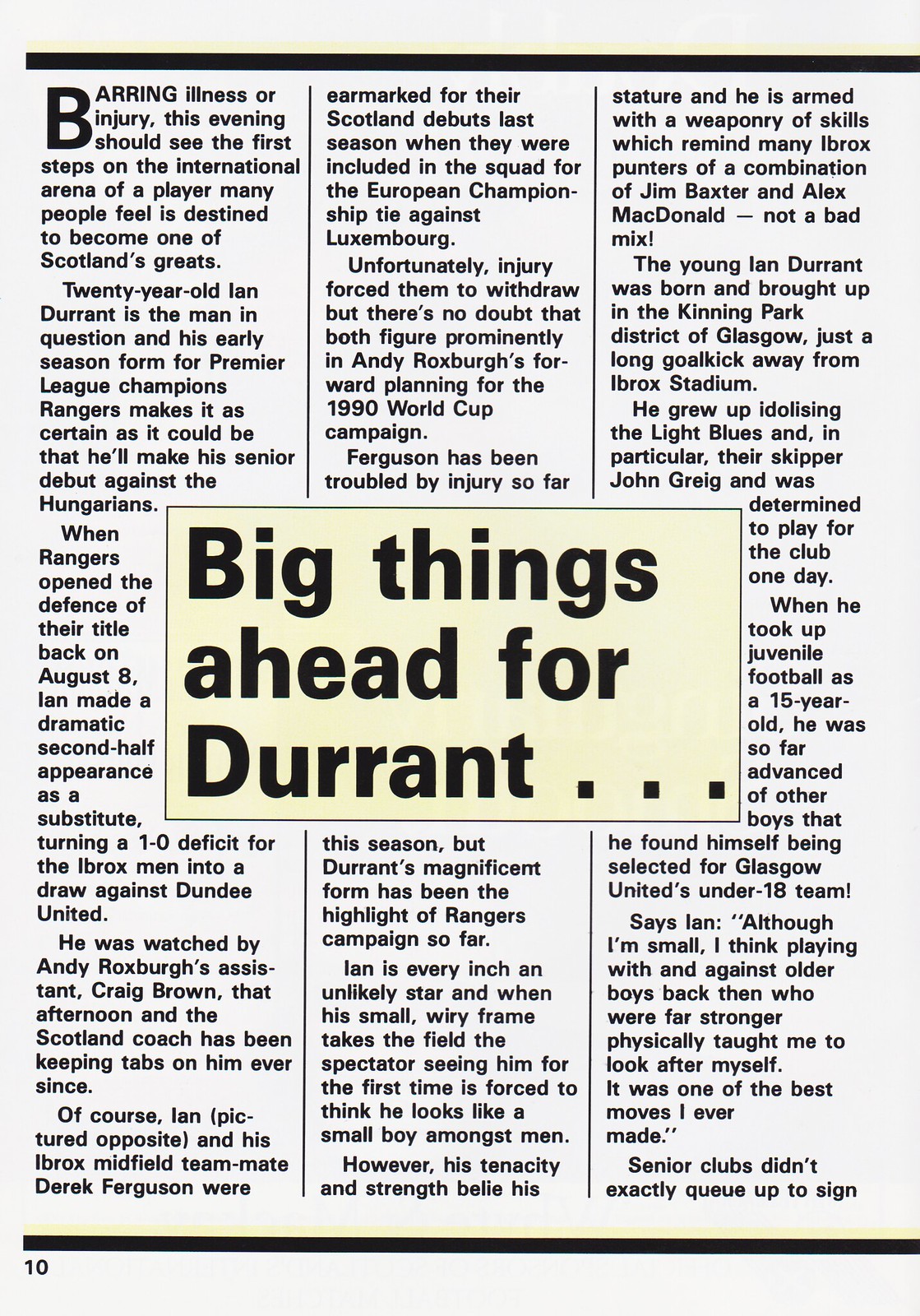A detailed black-and-white newspaper article on page 10, framed by black borders at the top and bottom, focuses on the promising career of 20-year-old Ian Durant. The headline reads, "Big Things Ahead for Durant," highlighting his potential breakthrough on the international stage. The article explores Durant's impressive early-season form for the Premier League champion Rangers, suggesting he is poised to make his senior debut against Hungary, barring illness or injury. Notably, Ian made a significant impact during the Rangers' title defense on August 8th, transforming a 1-0 deficit into a draw against Dundee United as a substitute, under the keen watch of Craig Brown, assistant to Andy Roxborough. Furthermore, both Durant and his Ibrox midfield teammate, Derek Ferguson, were considered for their debuts for Scotland in the previous season's European Championship tie against Luxembourg. Despite the lack of images, the text vividly portrays Durant's rising football career and his growing reputation as a budding Scottish football talent.